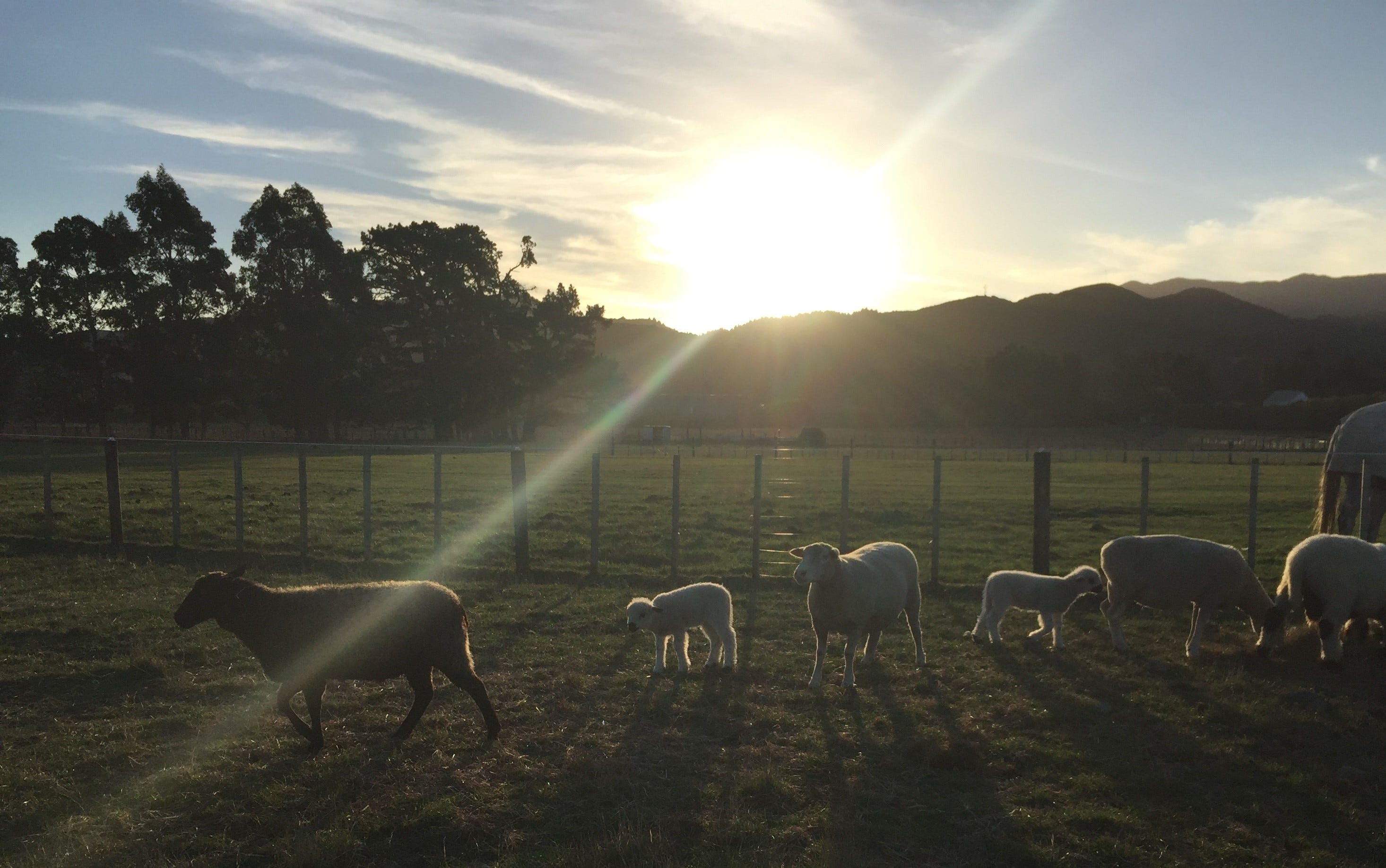In this picturesque photograph taken at sunset, a serene farm scene unfolds with a group of sheep and a solitary brown donkey within a fenced pasture. The black wire fence separates the foreground where three adult sheep and two lambs, all white, graze on patches of green and brown grass. The bright, setting sun casts a warm glow, creating a striking contrast that silhouettes the distant hills and accentuates the blue sky filled with beautiful clouds. The sheep on the right appear to be eating, while those on the left seem to be moving away. The background is adorned with lush trees and the majestic, green mountains, adding to the tranquil and scenic ambiance of this pastoral landscape.